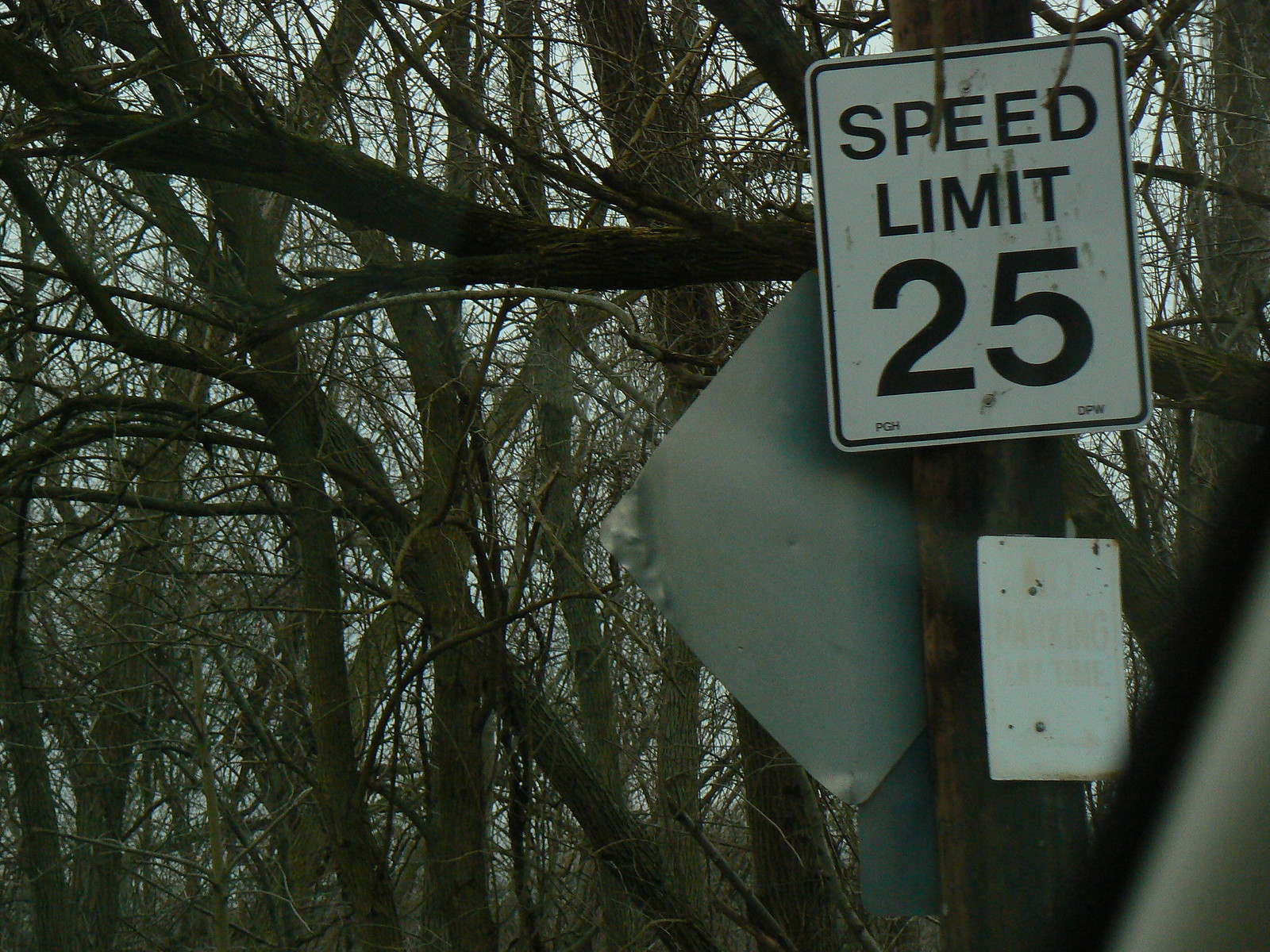The detailed image showcases a late evening or early morning scene at the edge of a wooded area. The sky is a muted light blue, almost white, with no direct sunlight filtering through. Dominating the scene is a web-like network of brown branches and twigs, creating an intricate, somewhat dark canopy. On the right side of the image, a standard white square street sign stating "Speed Limit 25" in black lettering stands prominently. Behind and slightly to the left of this main sign, there is the back of a gray, diamond-shaped traffic sign, its edges appearing beveled and bent. This forms part of a cluster of signs mounted on a single post, though only partial views of them are visible. The complexity of trees and branches envelops the scene, emphasizing the untamed nature of the surroundings.